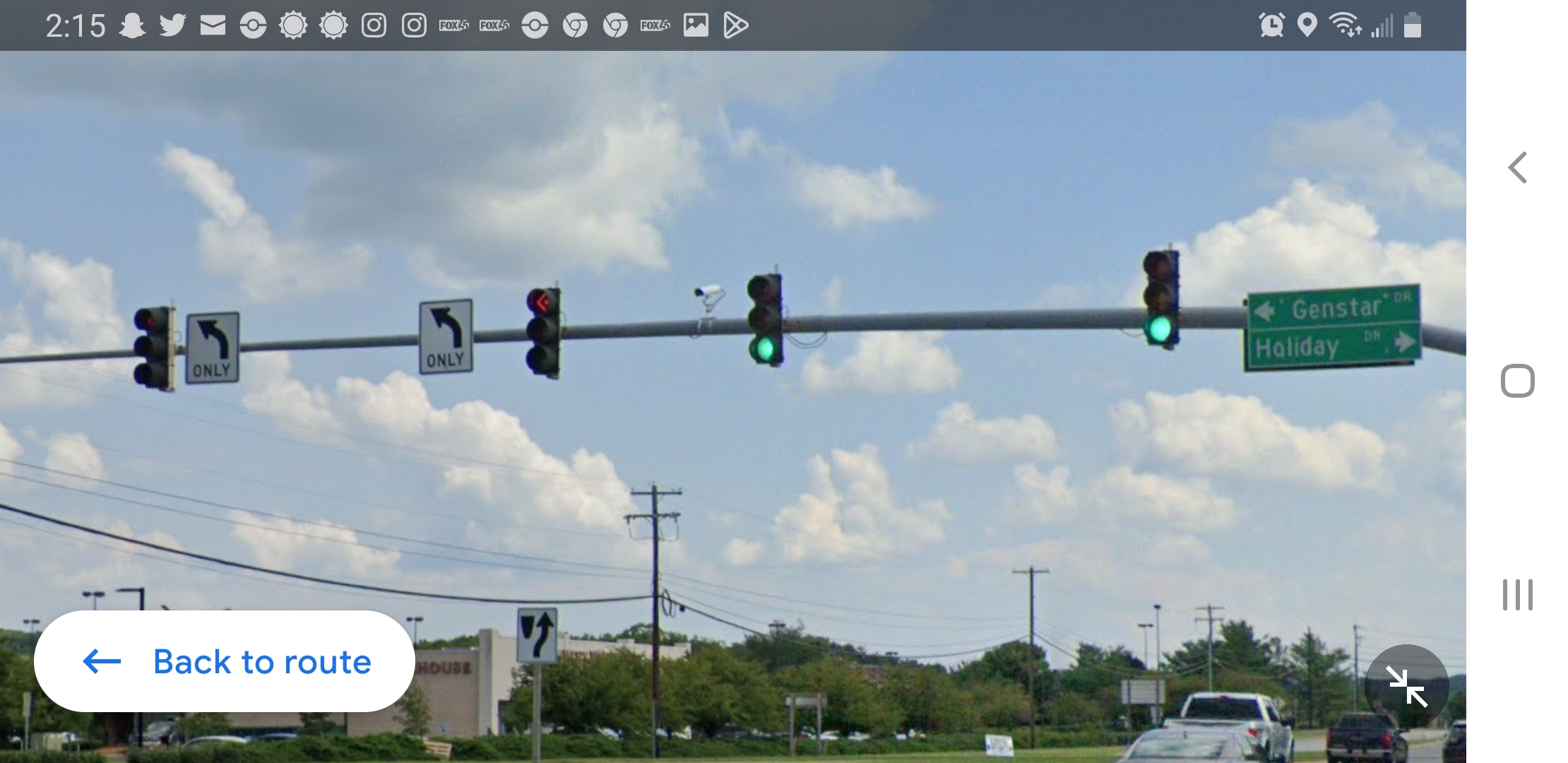This is a detailed screenshot taken from a phone, displaying a viewpoint that appears to utilize a map app in street view mode. At the very top of the image is the phone's menu bar, where the time indicates 2:15, and various icons and notifications are visible. Among the notifications are alerts from Twitter, email, Pokemon Go, AccuWeather, Instagram, Chrome, and the photo gallery. The phone's battery level is shown at half charge.

The main portion of the screenshot captures a busy intersection beneath a clear blue sky filled with many clouds. Central to the image is a tall pole bearing four stoplights and a traffic camera. The intersection's traffic lights include two green signals for straight travel and two red turn signals. Affixed to the pole are street signs indicating directions: "Genstar" to the left and "Holiday" to the right. Below these lights and signs, a green street sign further confirms the directional guidance.

On the lower part of the screen, a row of power lines can be seen running parallel to the road, which is lined with trees on one side. To the left side of the intersection, a beige building is partially visible, featuring a rectangular sign on its roof that reads “Back the Route” with an arrow pointing left.

In the lower right-hand corner of the photo, several cars and trucks are parked in a parking lot, adding to the detailed ambiance of this intersection scene.